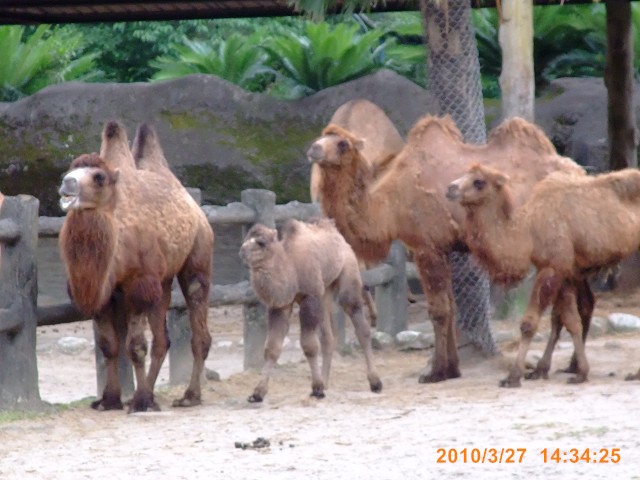This detailed photograph, likely taken at a zoo with an older digital camera, captures a group of four Bactrian camels standing and slightly facing to the left as if walking in unison. In the foreground, there's a wooden fence that runs from left to right, slightly shorter than the camels. The first camel, a brown adult with two humps, stands facing left. Adjacent to this camel is a lighter brown baby camel with a small developing hump, also looking left. Behind them are two more brown adults, both facing left, with one slightly smaller and with less pronounced humps.

The background features a tree line with bright green foliage and several trees, one of which is partially enclosed with a metal chain-link grating around its trunk. In front of the trees, there is a large, dark gray rocky area with hints of dark green algae or overgrowth. The ground beneath the camels is sandy, interspersed with patches of dirt and even some visible feces. In the bottom right corner of the photograph, a timestamp reads "2010-3-27 14:34:25," adding a specific historical context to the scene.